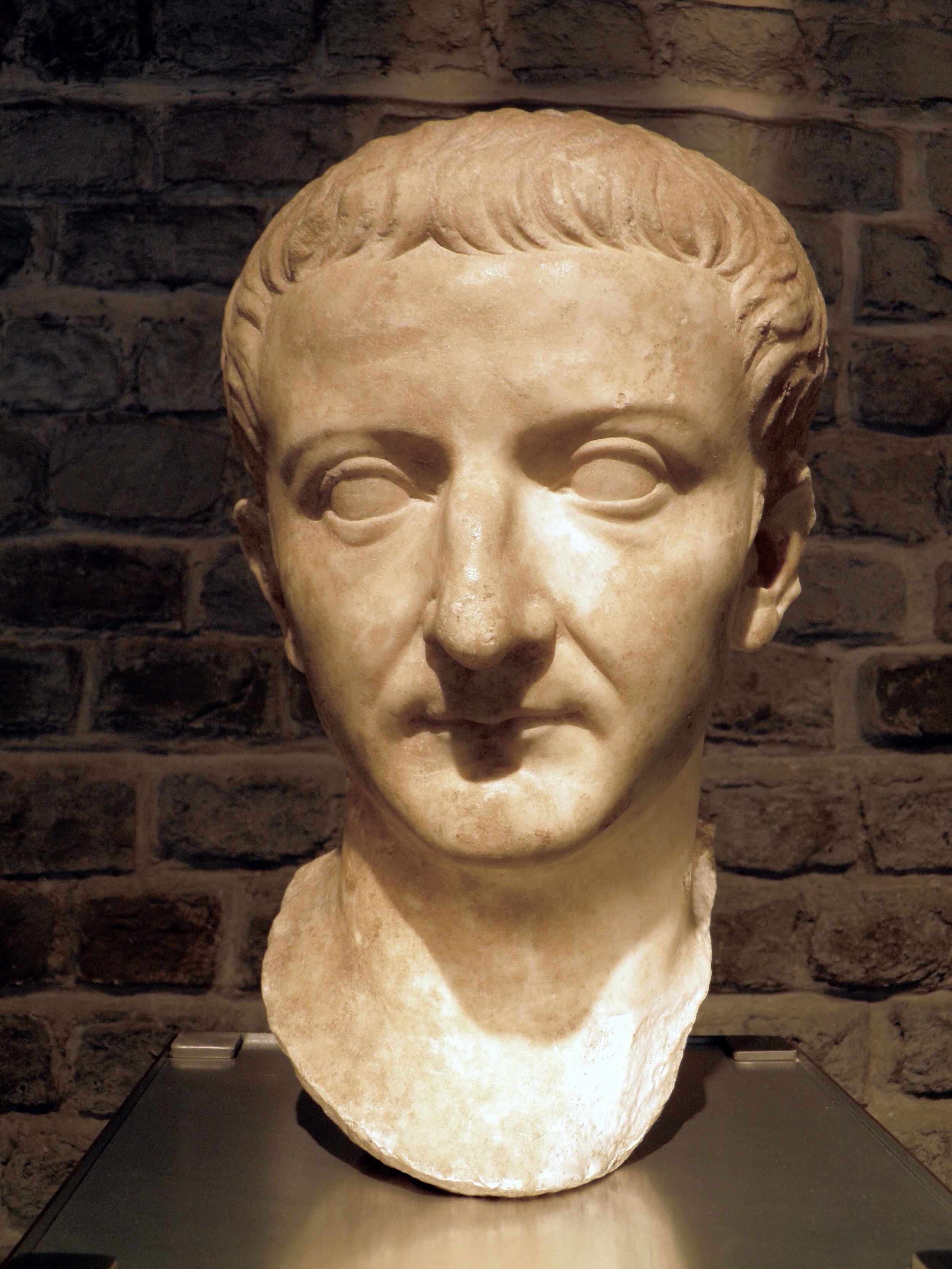This detailed bust appears to be an ancient marble sculpture, reminiscent of Roman or Greek artistry. Depicting a man from the neck up, the finely carved figure showcases very short hair with slightly wavy, forward-combed bangs. The face is marked by blank, pupil-less eyes giving it a strikingly eerie expression, a prominent, slightly bumped nose, and a small, calm mouth. The overall expression is neutral, lacking any evident emotion. The craftsmanship is preserved impeccably, showing no signs of wear or damage. Placed on a silver plate, the bust is situated before a backdrop of aged, dark brown bricks, hinting at a long history. The light source illuminates the statue, casting it in a dignified spotlight, emphasizing the man’s features and the refined quality of the marble. Despite the possibility that it could represent Julius Caesar or a similarly significant historical figure, the identity of the subject remains undefined. The entire setup rests on a metal table with visible posts at the corners, enhancing the classical and somewhat solemn ambiance of the display.